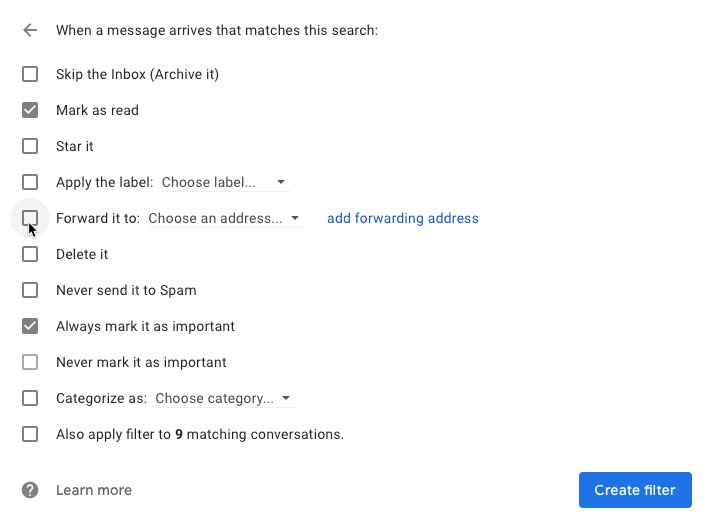**Detailed Caption:**

The screenshot captures a settings page from a website or application, featuring a pristine white background. In the top left corner, there is a medium gray arrow pointing to the left, immediately followed by a line of medium gray text stating, "When a message arrives that matches this search:". Below this line, there is a vertical array of checkboxes with dark gray outlines, each accompanied by specific text instructions.

1. The first checkbox is labeled "Skip the inbox (Archive it)".
2. The second checkbox is selected, filled with gray, and has a white checkmark in the center. It is labeled "Mark as read".
3. The third checkbox is labeled "Star it".
4. The fourth option reads "Apply the label:" followed by light gray text that says "Choose label" with a thin light gray underline and a black down-arrow indicating a dropdown menu.
5. The fifth option states "Forward it to" with a similar dropdown menu saying "Choose an address". Adjacent to this dropdown, there is blue text stating "Add forwarding address". There is a light gray circle around the checkbox on this line, and a black cursor with a white outline points to the checkbox.

Following these selections:

6. "Delete it".
7. "Never send it to Spam" (with "S" in "Spam" capitalized).
8. Another selected checkbox reads "Always mark it as important".
9. The next option with a light gray outlined checkbox says "Never mark it as important".
10. "Categorize as:" followed by a dropdown menu reading "Choose category...".
11. The final option states "Also apply filter to 9 matching conversations," with the number nine bolded and black.

In the bottom right corner of the screenshot, there is a prominent blue button with white text that says "Create filter".